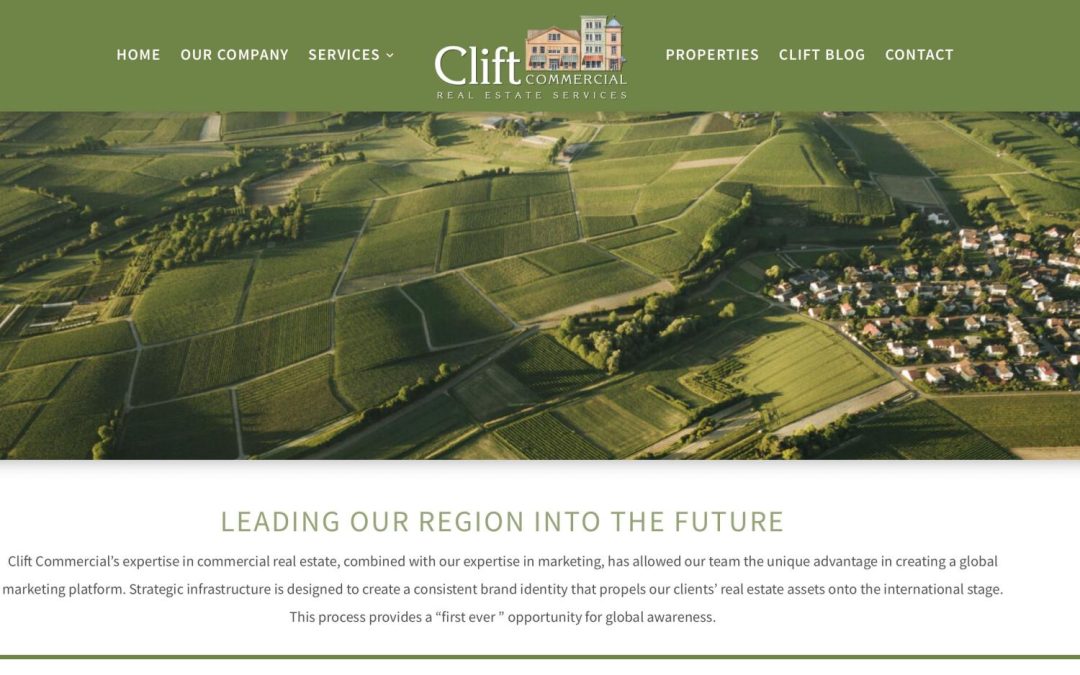The image is a screenshot of a professional website, dominated by a serene green landscape with neatly organized sections of mowed grass. To the right of the image, a quaint residential community with various small houses is visible, nestled beside vast, manicured fields.

At the top of the website, a wide green header displays a white navigation menu that includes "Home," "Our Company," "Services," "Properties," "Clift Blog," and "Contact," with some options featuring a drop-down menu icon. Centrally positioned within the header is the Clift Commercial Real Estate Services logo, depicted with white text and a small image of three buildings.

Below the header, bold capitalized text reads, "LEADING OUR REGION INTO THE FUTURE." Beneath this slogan, a detailed paragraph in black text describes Clift Commercial's expertise in commercial real estate and marketing. It highlights the unique advantage of their global marketing platform, which creates a consistent brand identity and promotes their clients' real estate assets on an international scale, providing an unprecedented opportunity for global awareness.